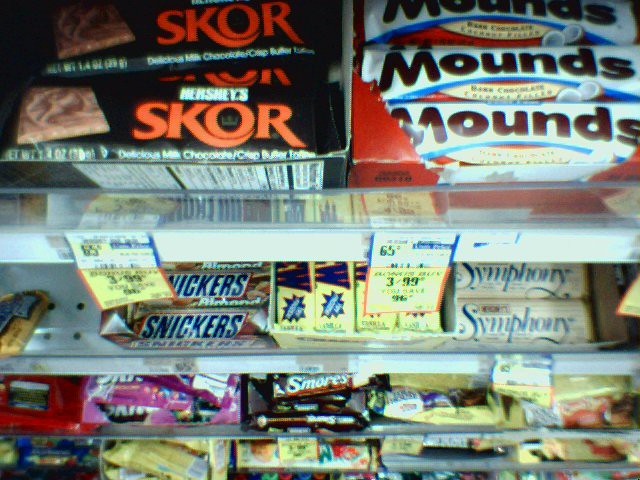This photograph captures a close-up view of an "Impulse Isle" or "Temptation Isle" at a grocery store, showcasing four shelves filled with a colorful array of candy and chocolate bars. At the top left, Hershey's Score bars are neatly placed, while Mounds bars, with their distinctive red and white wrappers, occupy the right side. Beneath these, Snickers Almond bars, and Hershey's Symphony bars are visible alongside Charleston Chews, discernible by the partial view of the "W" on their packaging. Price tags are prominently displayed, indicating prices of $3.93, $4.99, and 65 cents each. The next shelf down features a mix of s'mores and other indistinguishable but vibrant chocolates. The quality of the image blurs slightly on the lower shelves, where Peanut Butter M&Ms, possibly a Kit Kat, purple Skittles, a S'mores bar, Toll House cookies, and what might be a Carmelo Bang are stocked. The bottom row houses a mix of fruit candies, including Mambas, with some empty spaces and tan-colored candies that are difficult to identify. The overall scene is a tempting display of sugary treats, inviting shoppers to make a last-minute purchase.